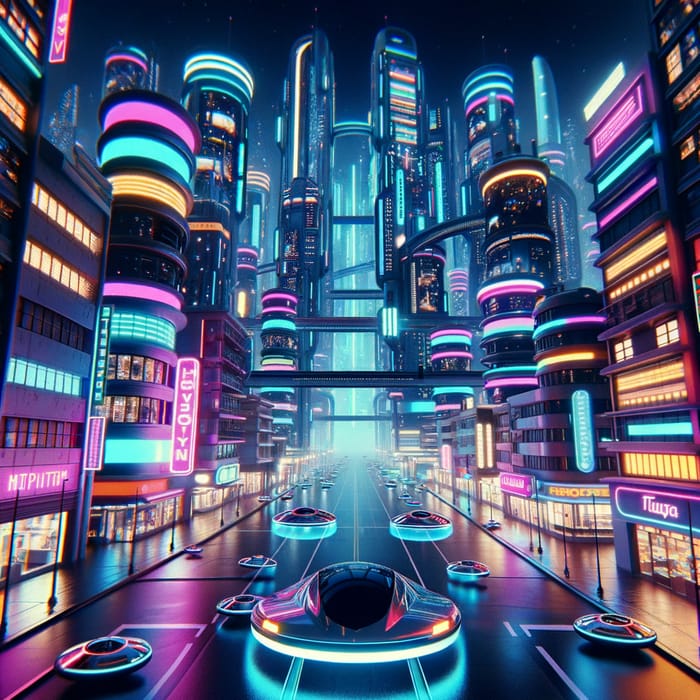The image depicts an AI-generated futuristic cityscape bursting with vibrant neon colors, set against a dark blue night sky. The scene is filled with towering, cylindrical skyscrapers that are adorned with rings of magenta, cyan, and yellow lights, creating an almost otherworldly ambiance. Some of the buildings feature signs with indecipherable text in a strange language, adding to the futuristic allure. The meticulously clean sidewalks and streets are dotted with round, hover cars emitting bright blue lights from their undercarriages, gliding seamlessly at various heights above the ground. In the middle of the urban tableau, bridges connect the buildings, reminiscent of a bustling, high-tech version of Las Vegas. The overall illumination from the brightly lit buildings casts a radiant glow onto the roads and sky, enhancing the mesmerizing and hyper-modern atmosphere of this city of the future.